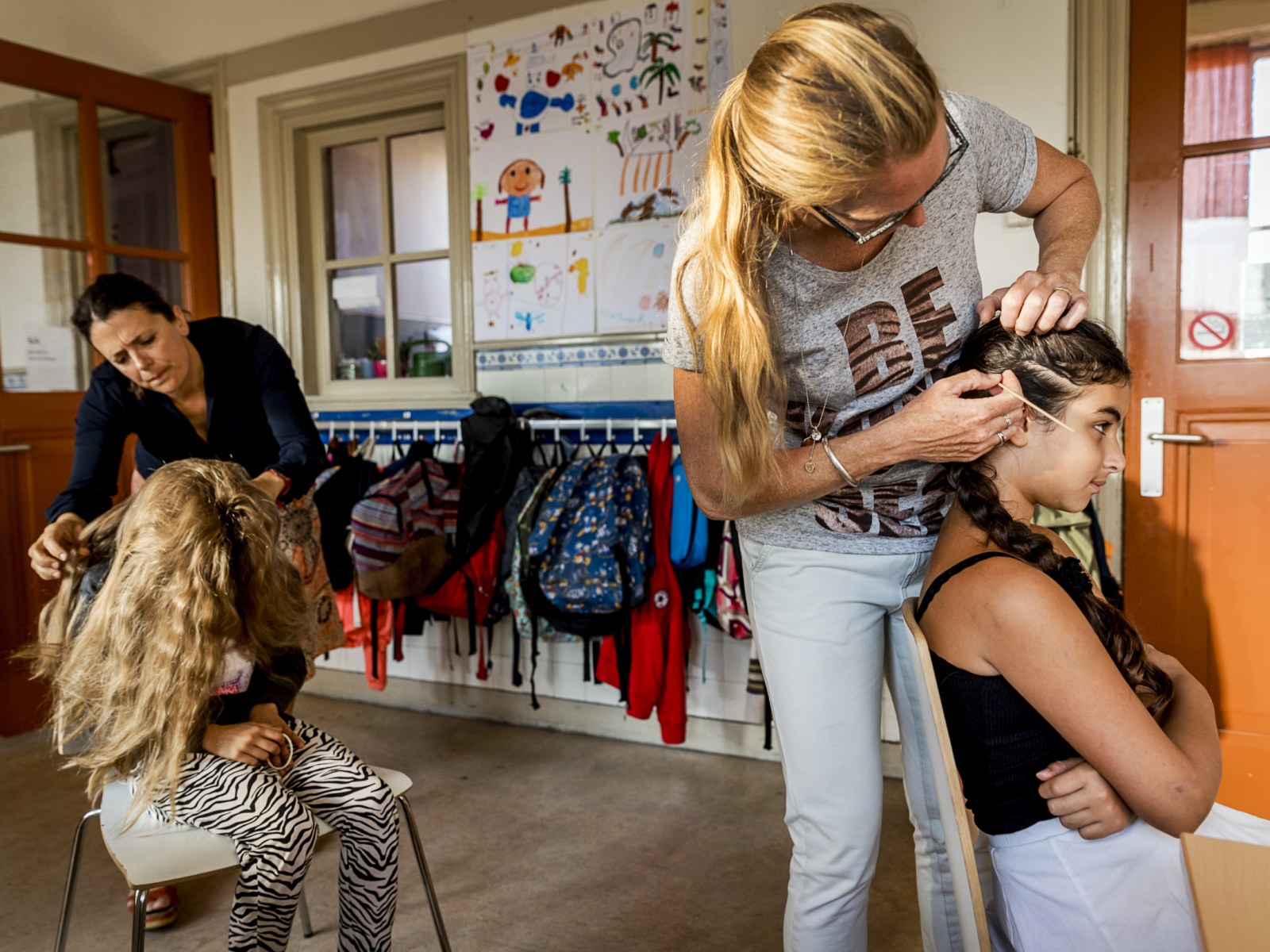In this image, two young girls, appearing to be around 8 to 12 years old, are seated in a room that resembles a classroom or an after-school care area. The room's back wall is lined with hooks holding various backpacks and jackets, and there are brown doors in both the left and right corners. Both girls are having their hair inspected, likely for lice.

The girl on the left is wearing zebra-patterned pants and a black shirt, with her light brown hair tipped forward as a woman in a black long-sleeve shirt with dark hair leans over her, carefully checking her hair. The girl on the right has long dark hair, a black tank top, and white bottoms. Another woman, wearing glasses, a gray short-sleeve shirt with lettering, and light-colored jeans, is also leaning over, inspecting this girl's hair. The atmosphere suggests a thorough examination, typical of a school lice check.